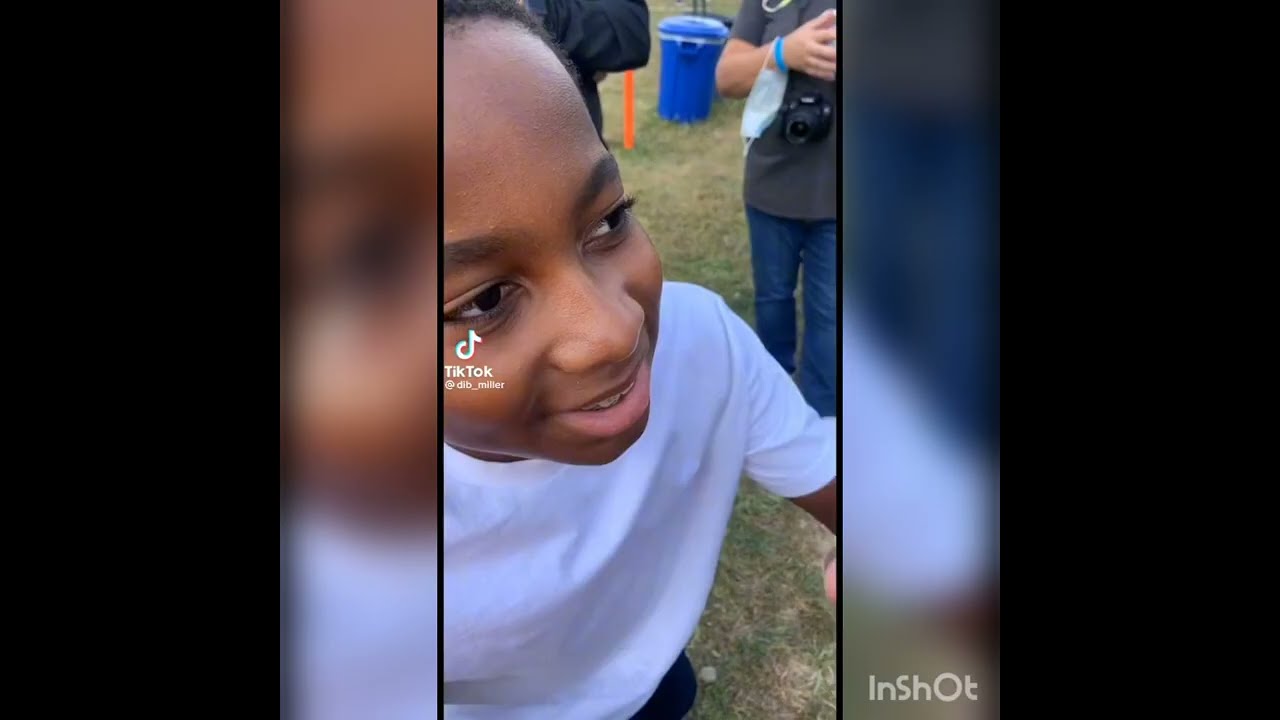The image depicts a young black boy with short hair and braces, standing on the left side of the frame and facing to the right with a slight smile. He is wearing a white short-sleeved t-shirt and black pants, with part of the pants visible at the bottom of the image. The boy is in a grassy field, and behind him, there is another person, partially visible, wearing a gray short-sleeved t-shirt and blue jeans. This person is holding a black camera and has a blue temporary wristband on their wrist. In the background to the right, there is a medium-sized blue cylindrical trash can. The scene also includes some minor details like an orange pylon and part of a black jacket behind the boy’s head. The image appears to be a still from a TikTok video, indicated by the TikTok symbol and a handle, possibly reading "@DLO_Miller" or "@DLB_Miller". Additionally, the InShot text is present at the bottom right of the image, which implies it was edited using the InShot app. The color palette of the image includes brown, white, pink, green, tan, orange, blue, and gray.